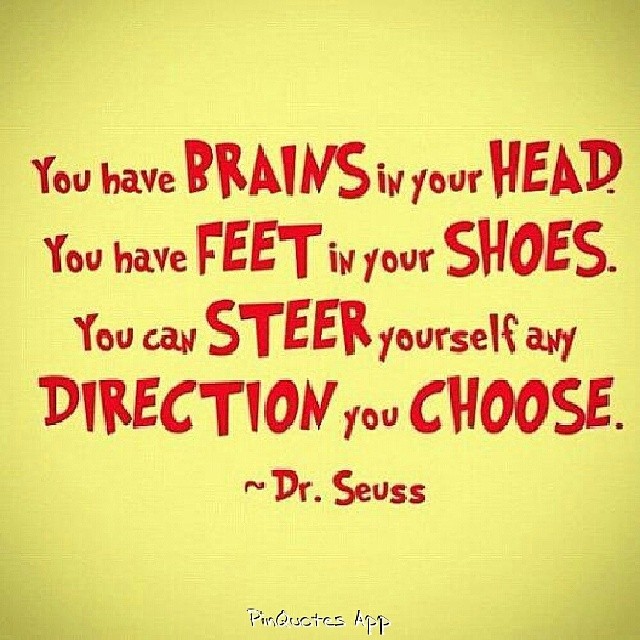The image features a fuzzy, artifacted style typical of a low-resolution JPEG, with a Dr. Seuss quote displayed prominently. The background is a light yellowish-green hue, and the text is predominantly red, while a small white text at the bottom indicates "pin quotes app." The quote reads: "You have brains in your head. You have feet in your shoes. You can steer yourself any direction you choose." In the quote, the words "brains," "head," "feet," "shoes," "steer," "direction," and "choose" are capitalized and much larger than the surrounding text, which emphasizes their importance. The text is centered within the square image, creating a visually balanced layout. At the very bottom of the image, the attribution "Dr. Seuss" is signed off in smaller letters, aligning with the whimsical and motivational style characteristic of Dr. Seuss's books.